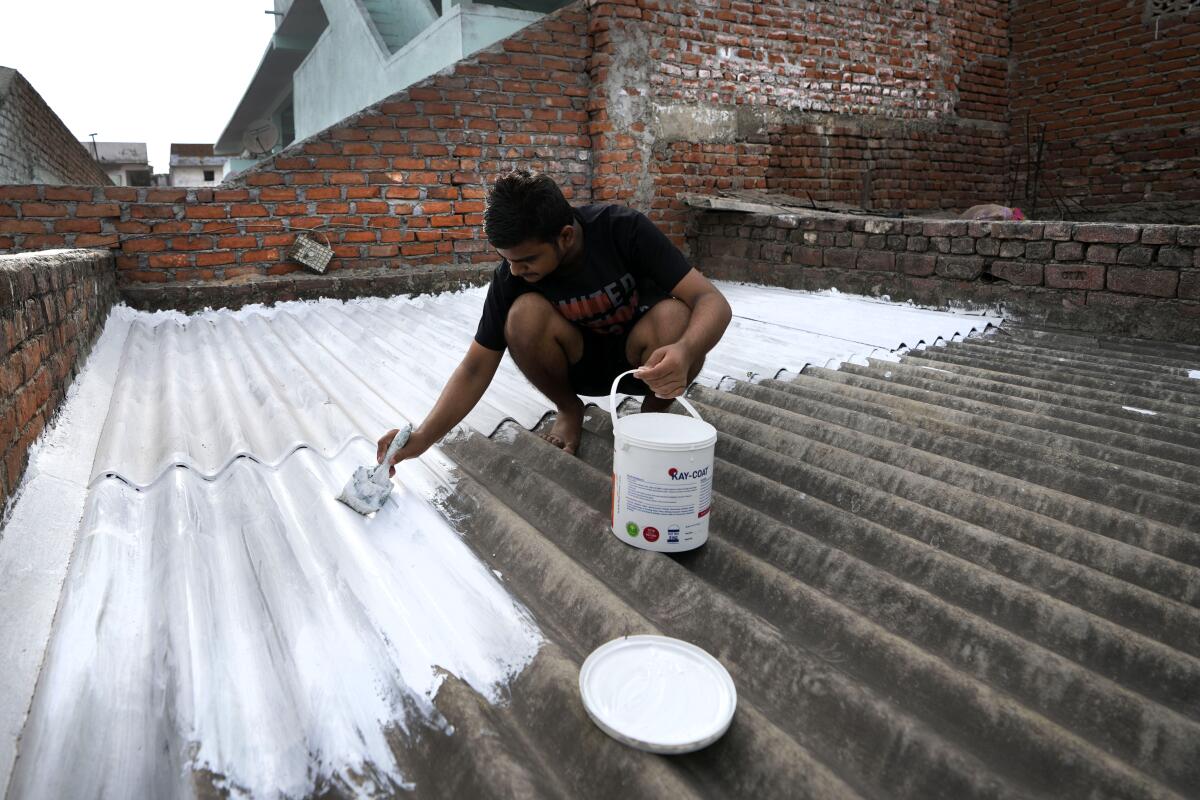The photo depicts a barefoot man dressed in a black T-shirt and black shorts, crouching on a corrugated metal rooftop and painting it white with a paintbrush. The can of white paint sits nearby, with its lid discarded to the side. The surroundings include aged, dirt-streaked brick walls where the mortar is visibly chipping away, indicating the rooftop is atop an older building, likely an apartment complex. The man appears to be enjoying his task, as he methodically applies the paint to the ribbed metallic surface, creating orderly lines. In the background, additional buildings can be seen, though they lack any distinctive features.